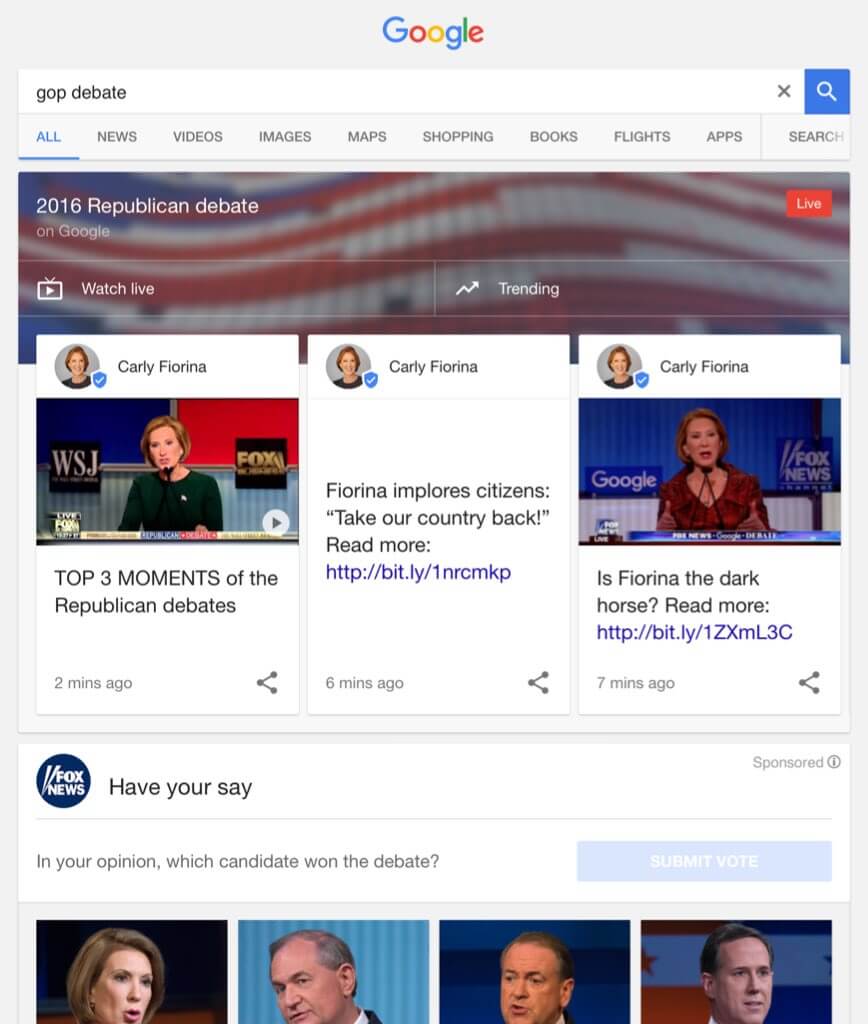A detailed descriptive caption for the provided image would be:

"The image shows a gray-background screenshot of Google search results for 'GOP debate'. At the top, the search bar contains the query 'GOP debate'. Below the search bar, there's a horizontal menu providing options for different types of search results, including 'All' (selected), 'Videos', 'Images', 'Maps', 'Shopping', 'Books', 'Flights', 'Apps', and 'News'. The main content area features a dominant section titled '2016 Republican debate', primarily occupying the central part of the screen. Immediately beneath this title, there's a banner announcing 'Dollar fonts on Google'. Following this, two horizontal bars are visible: one labeled 'Watch live' and the other 'Trending', both displayed against a vaguely blurred American flag backdrop. Below these bars are three side-by-side blocks. The first block highlights 'Top three moments' from Carly Fiorina, while beneath these blocks, there's a prompt encouraging user interaction that reads, 'Have your say'."